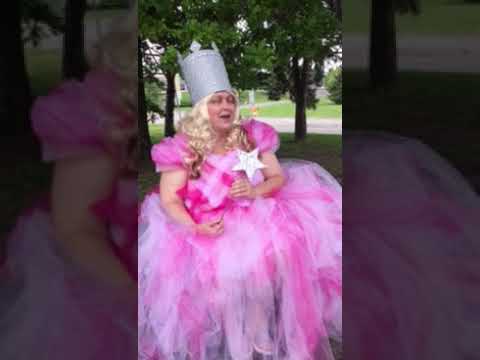An adult, possibly male, dressed as a fairytale or Disney princess stands in a shadowed park area with two large trees and some buildings visible in the background. They are wearing an elaborate, extremely frilly pink and white dress with puffed shoulders and a diagonally patterned bodice. Their outfit includes a tall, metallic-looking crown that appears to be made of either plastic, wood, or paper, and a long, blonde wig. In their hand, they hold a wand topped with a shiny, sparkly star. The individual is looking off to the right, seemingly in response to something out of the frame.